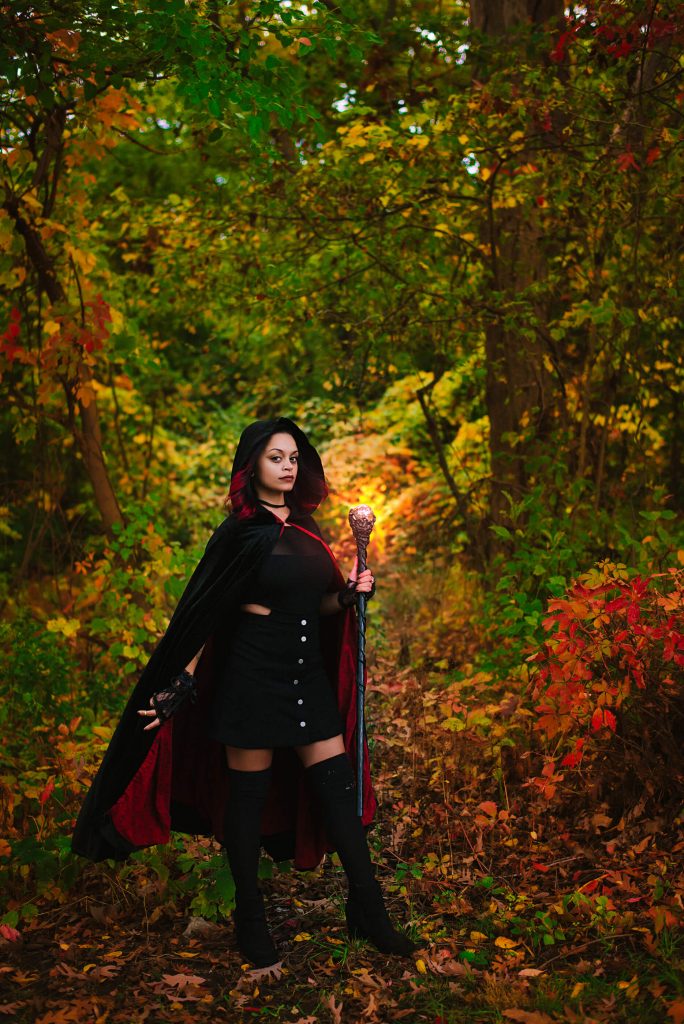In this outdoor photograph set during early autumn, a woman stands amidst a forest backdrop rich with yellow, red, and green leaves. The ground beneath her is carpeted with fallen foliage, adding to the seasonal atmosphere. She is dressed in elaborate cosplay-like attire, evoking the image of a sorceress. Her outfit features a long black cloak with a dark red, likely velvet, lining. She wears a short black dress adorned with white buttons down the middle, paired with thigh-high black lace gloves and black boots with a slight heel. Her black hair contrasts against her fair skin, which has a slightly darker tone. Around her neck is a black choker necklace. In her hand, she holds an ornate staff, the shaft appearing blue metallic with a golden orb at the top, completing her mystical ensemble.